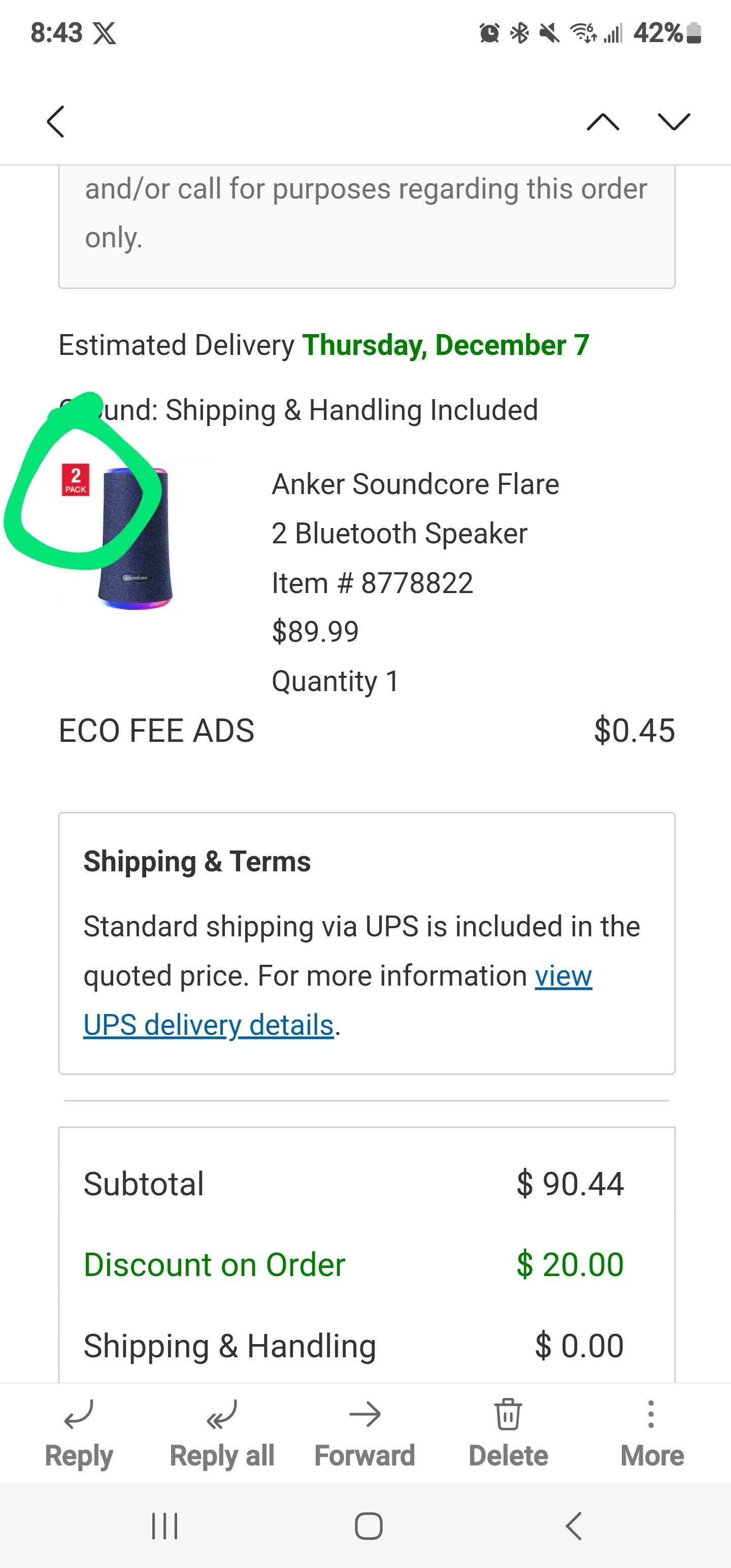A detailed screenshot of a mobile email confirmation for an order of the Anker Soundcore Flare 2 Bluetooth speaker. At the top, there's a text box stating "and/or call for purpose regarding this order only." The estimated delivery is noted as Thursday, December 7th, with ground shipping and handling included. The ordered item is the Anker Soundcore Flare 2 Bluetooth speaker, item number 8778822, priced at $89.99 with a quantity of 1. There is an EGO fee of $0.45. 

To the left of the product description, there is a blue speaker image with a prominent green circle drawn around a red box that indicates the number "2." Below this section, another box mentions that standard shipping by UPS is included in the quoted price, with an option to view more details about UPS delivery, highlighted in blue text. 

The subtotal is $90.44, from which a $20 discount is applied (highlighted in green), making the final total for shipping and handling $0.00. 

At the bottom of the screenshot, typical email interaction buttons are visible, including "Reply," "Reply All," "Forward," "Delete," and "More." The top right corner of the screenshot shows the phone's battery is at 42% with a timestamp of 8:43 AM, and there is an "X" notification icon.